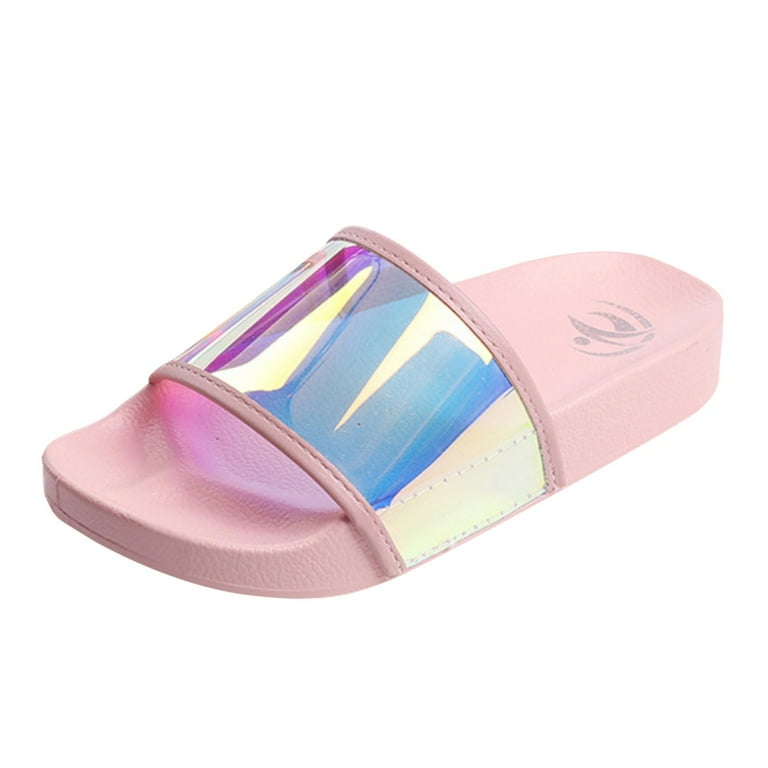This image features a single light pink slip-on sandal with a thick, foam-like, cushioned sole that has grooves designed for added grip. The sandal is set against a complete white background and is angled with the toe part facing the bottom left corner. The standout feature is the sheer, reflective strap that arcs over the toes, displaying a rainbow-like sheen with hues of pink, purple, and blue. This strap is bordered by sewn-on pieces of pink leather on each side. Additionally, the heel section inside the sandal showcases a grayish-black image of a person jumping, adding a subtle design element to the footwear. The overall aesthetic combines comfort with a stylish, reflective detail that catches the light beautifully.